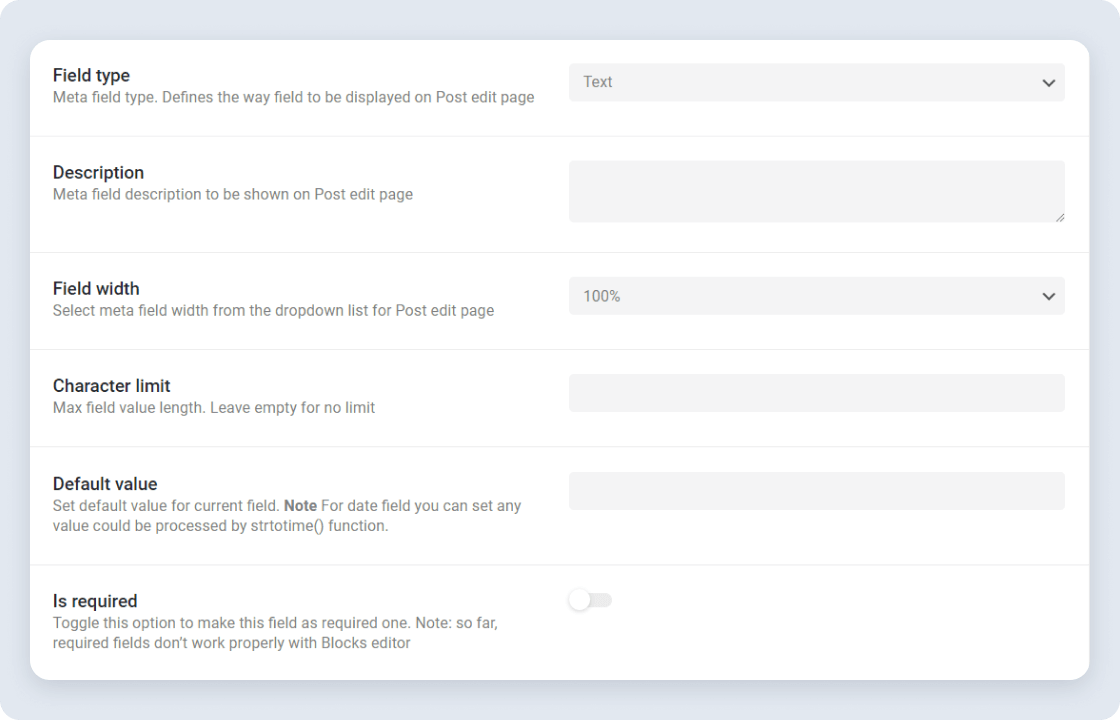Screenshot of a website form with a white background, possibly a pop-up blocking the underlying webpage. The form appears to be part of a website builder tool, as suggested by the structured layout and field descriptions. 

On the left side, labels for various meta fields are listed:
1. **Field Type**: Describes the format in which the field will appear on the post edit page. To the right, there is a drop-down menu for selecting the field type.
2. **Description**: Specifies what the meta field description will show on the post edit page, accompanied by a text input field for user input.
3. **Field Width**: Allows users to choose the width of the field via a drop-down menu.
4. **Character Limit**: A text input field where users can set the maximum number of characters allowed.
5. **Default Value**: Another text input field for specifying a default value for the field.
6. **Is Required**: Features a toggle switch to mark the field as required. 

A note at the bottom reads: "So far, required fields don't work properly with Glocks editor."

Each field type and description is designed for ease of form customization, enabling users to configure how information is displayed and managed on their website's post edit page.